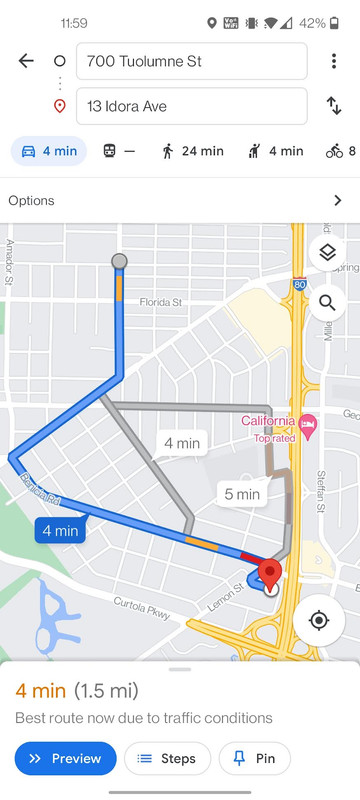The image displays a Google Maps navigation screen showing directions to a destination. The current time is 11:59 PM, clearly visible at the top of the screen. In the upper right corner, several status icons are displayed, including Wi-Fi, cellular reception, battery at 42%, and the battery icon.

The navigation interface includes fields indicating the starting point and destination. The start location is listed as "70020 Lume Street," and the destination is "13 Edora Avenue." Below these fields, various transport options are depicted with corresponding travel times. A car icon indicates a 4-minute journey in blue, whereas a train icon is shown with a dash, likely indicating that train travel is not available or applicable. Next to the train icon, a walking figure suggests a 24-minute travel time. A taxi icon, represented by a character raising their arm, shows a 4-minute travel time, and lastly, a cyclist icon indicates an 8-minute journey.

The map itself features a prominently displayed blue path, signifying the recommended route. This path starts with a gray marker and ends with a red marker, indicating the start and finish points, although this might be reversed. The blue path is labeled with a travel time of 4 minutes. There are also alternative paths highlighted in gray with travel times of 4 and 5 minutes. The map prominently displays streets such as Florida Street.

Beneath the map, text indicates that the 4-minute, 1.5-mile route is currently the best option due to traffic conditions. Three action buttons are presented at the bottom: a blue "Preview" button, a white "Steps" button, and another white button labeled "Pin" with a small blue pin icon.